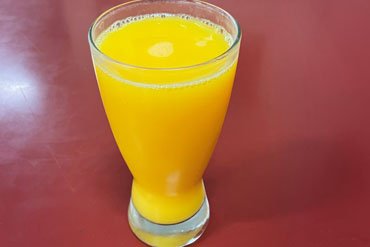Centered in the photograph is a tall, clear Pilsner-style glass filled with bright yellow-orange juice, possibly fresh orange juice with pulp. The glass is set on a burgundy or red countertop, which exhibits signs of wear and tear, adding character to the setting. The juice fills the glass to within about 20 millimeters of the rim, and there's a layer of tiny bubbles and foam around the edge, suggesting it was recently poured. The glass has a narrow base that gradually widens to a broad top, creating a flowing, curvy shape. Positioned under a light source, likely a camera flash, the left side of the image is slightly illuminated, giving a subtle highlight to the scene. The overall composition is simple and minimalistic, focusing solely on the refreshing glass of juice.